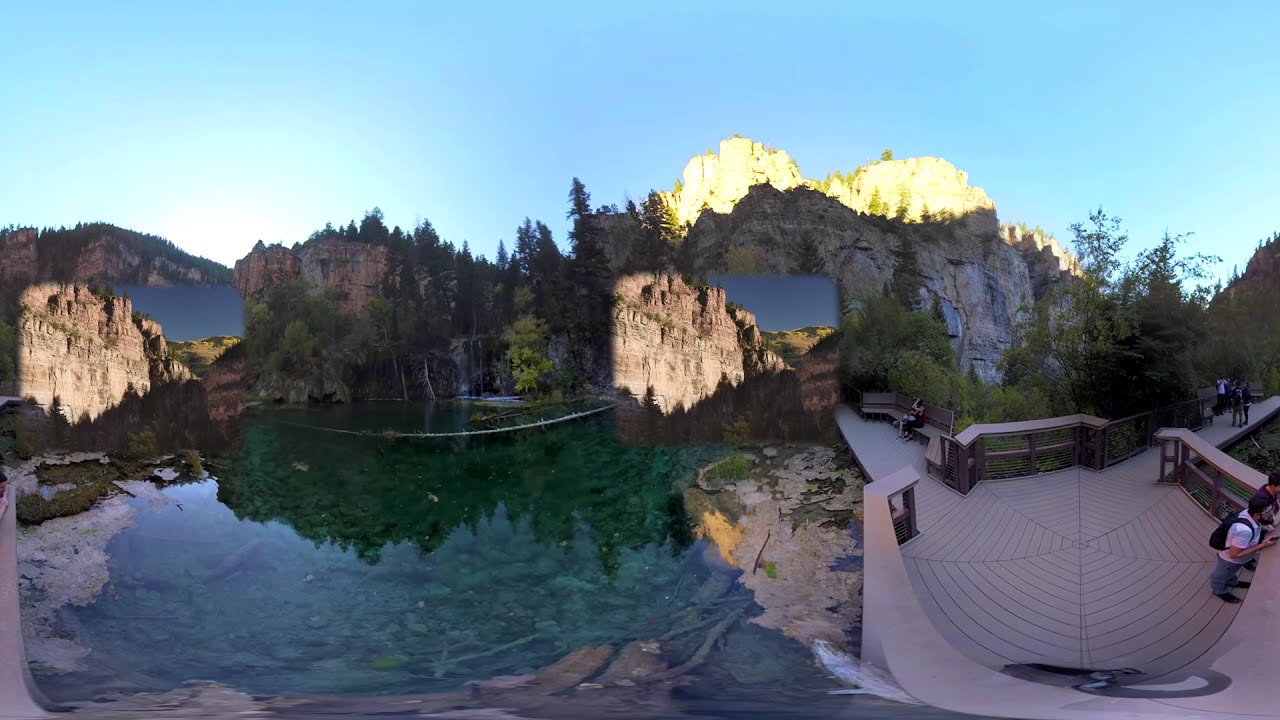The image captures a breathtaking mountain scene set within a park, featuring a crystal-clear lake with a bluish-green tint nestled in the center-left. The lake's still waters beautifully reflect the surrounding tall pine trees and jagged granite mountains. On the right-hand side of the image, there is a wooden observation deck with railings and a safety berm, offering a panoramic view of the magnificent landscape. Two men wearing backpacks—one in a white shirt and jeans, the other in a black shirt with dark hair—stand at the edge of the deck, taking in the scenery. Other visitors can be seen walking, sitting, and mingling along the wooden boardwalk that connects to two pathways leading into the forested mountain area. The sky is a crystal-clear blue, and the atmosphere is serene, highlighting the natural splendor of the landscape.